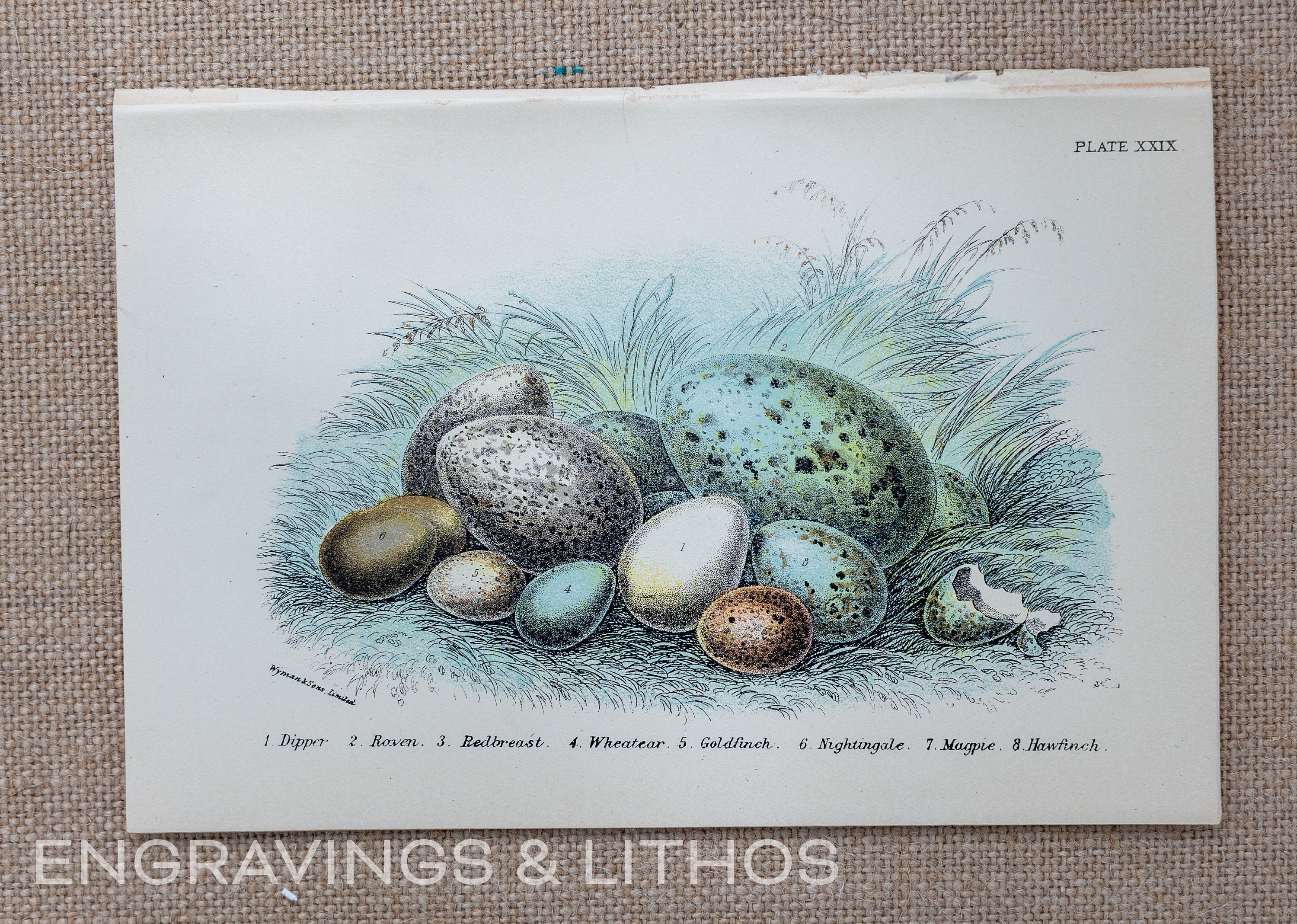This detailed photograph captures an illustration of various bird eggs, carefully arranged against a distinctly tan cork board background. The illustration, featuring a white backdrop, showcases eight different types of eggs, meticulously drawn and labeled: a dipper, a raven, a boldreast, a wheat ear, a goldfinch, a nightingale, a magpie, and a hawfinch. Notably, the image includes diverse colors and patterns, such as a large blue-green egg with black spots, a brown egg, a white egg with brown specks, and an orange egg with black specks among others. There are also eggs in shades of blue with specks, and plain white and brown eggs. Additionally, the top right corner bears the inscription "plate XXIX," and prominently at the bottom, in white lettering, are the words "engravings and lithos." The scene seems to be set outdoors in a patch of blue-green grass, framed by reeds and other plants, adding a rich, natural context to the assortment of intricately detailed eggs. There's also a notable broken eggshell in the bottom right, adding a touch of realism to the composition. The entire artwork appears mounted on material resembling a brown burlap sack, giving it a rustic feel.